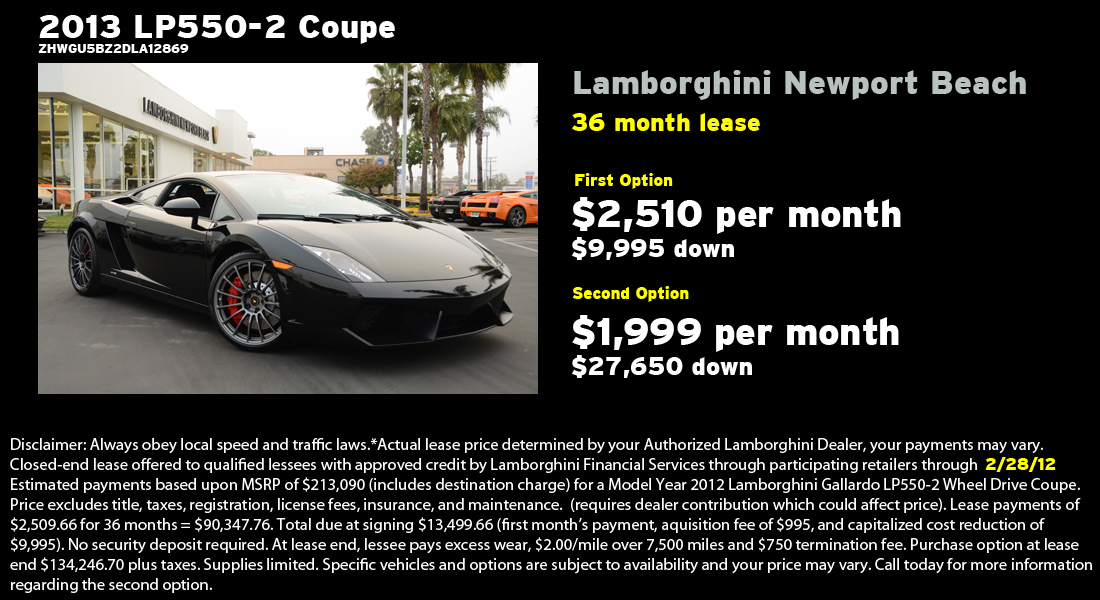The image is an advertisement for a 36-month lease on a 2013 Lamborghini LP 550-2 Coupe from Lamborghini Newport Beach. Set against a solid black background with predominantly white text, the ad is meticulously detailed. In the upper left corner, "2013 LP550-2 Coupe" is prominently displayed, accompanied by smaller text likely indicating the VIN number. Below this is a horizontally rectangular photograph of the sleek, black, two-door sports car featuring distinctive silver and red-decorated wheels.

To the right of the photograph, "Lamborghini Newport Beach" is written in light gray letters. Below this, in yellow text, it reads "36-month lease," followed by "first option" in smaller yellow text. The subsequent line in larger white print states "$2,510 per month," with fine print below it indicating "$9,995 down." Further down, another yellow line reads "second option," followed by "$1,999 per month" in larger white print, and "$27,650 down" in smaller white print.

At the bottom of the advertisement, there is a block of small, white text containing the lease agreement details, including that lease payments for the first option total approximately $90,000 and a purchase option at lease end of $134,246.70. Though difficult to read in the image, this text likely includes other important disclaimers and conditions.